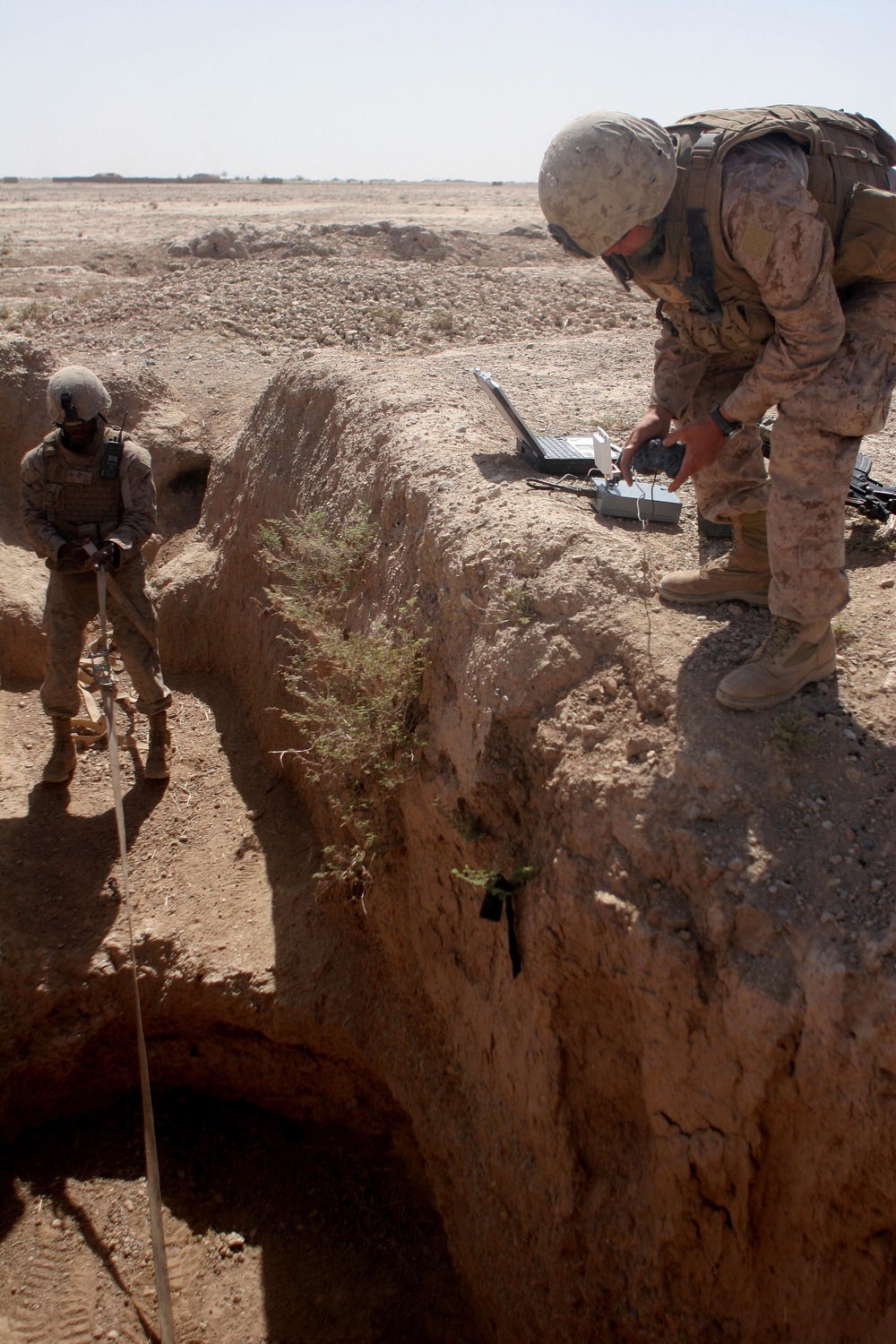In this image of a military combat exercise set in a vast, barren desert under a cloudless, pure blue sky, two soldiers in full camouflage gear are engaged in an operation involving a hole or cave. The floor of the desert is scattered with rubble, rocks, small gravel, and there are some trees and indistinct buildings visible in the top left of the image. The soldier on the left, dressed in a full khaki outfit with tan combat boots, protective helmet, and armor, is positioned lower, at the edge of the hole, holding onto a rope or similar material, suggesting he may be lowering or retrieving something. Meanwhile, the soldier on the right stands on a rocky ridge above, focused on his laptop and holding a controller, seemingly measuring or pinpointing something based on data. Both soldiers are equipped with vests, walkie-talkies, and other standard military gear, conducting their operation against a backdrop of endless desert.